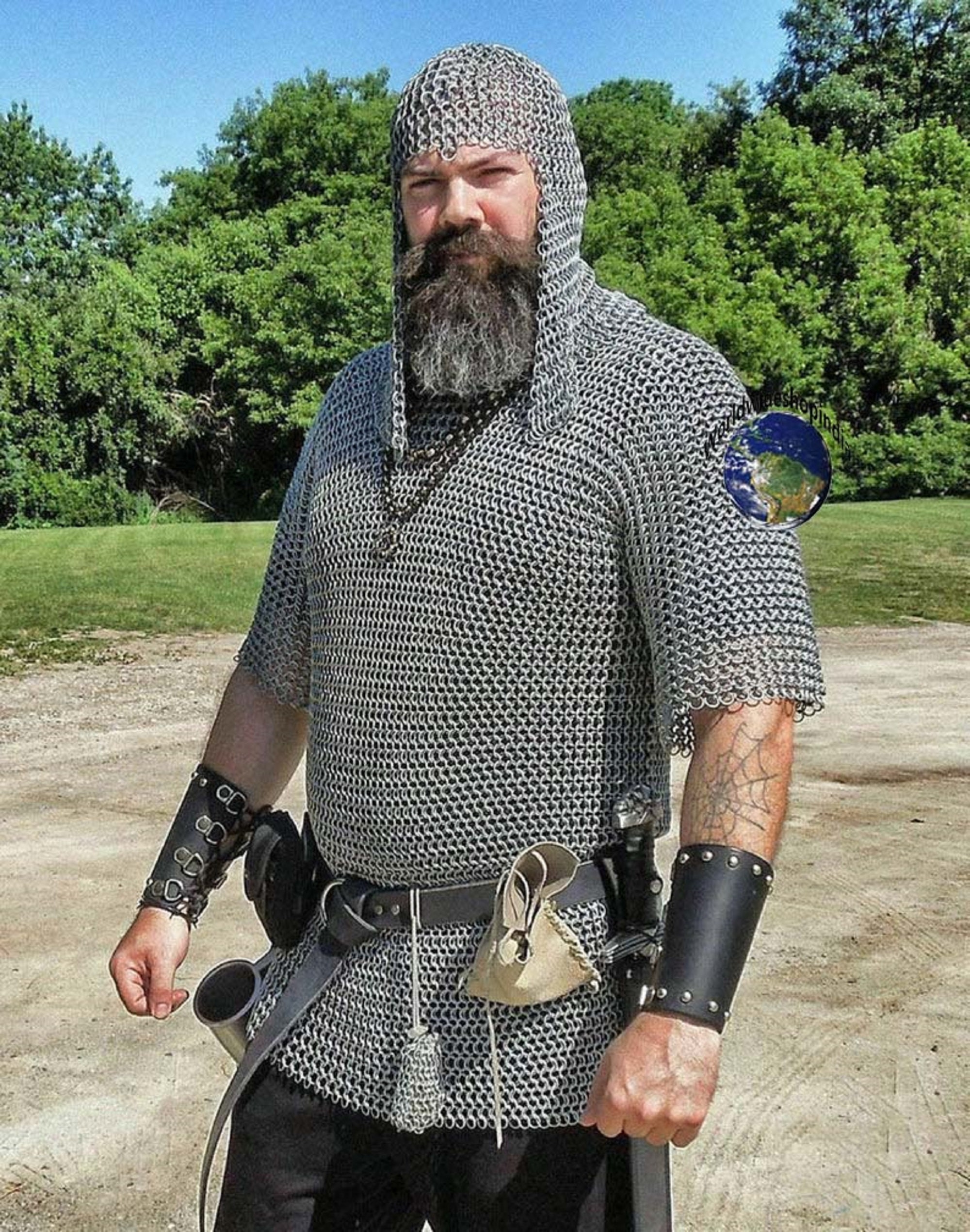In the photo, a white-skinned man with a long gray beard is seen standing outdoors on a light dirt road amidst a background of green trees, bushes, and grass. The blue sky suggests it is daytime. He is dressed in elaborate medieval armor, likely for a reenactment or cosplay event. His outfit includes a full chainmail shirt that covers his torso and a chainmail coif that extends down beyond his neck for added protection. A large silver chain hangs around his neck, and a well-worn black leather belt with various attached items, including a small bag and possibly a knife, cinches his waist. Black leather wrist guards and black pants complete his ensemble. There is also an intriguing overlay of a planet with the text "World Wide Shop Indy," likely indicating the retailer of his costume.